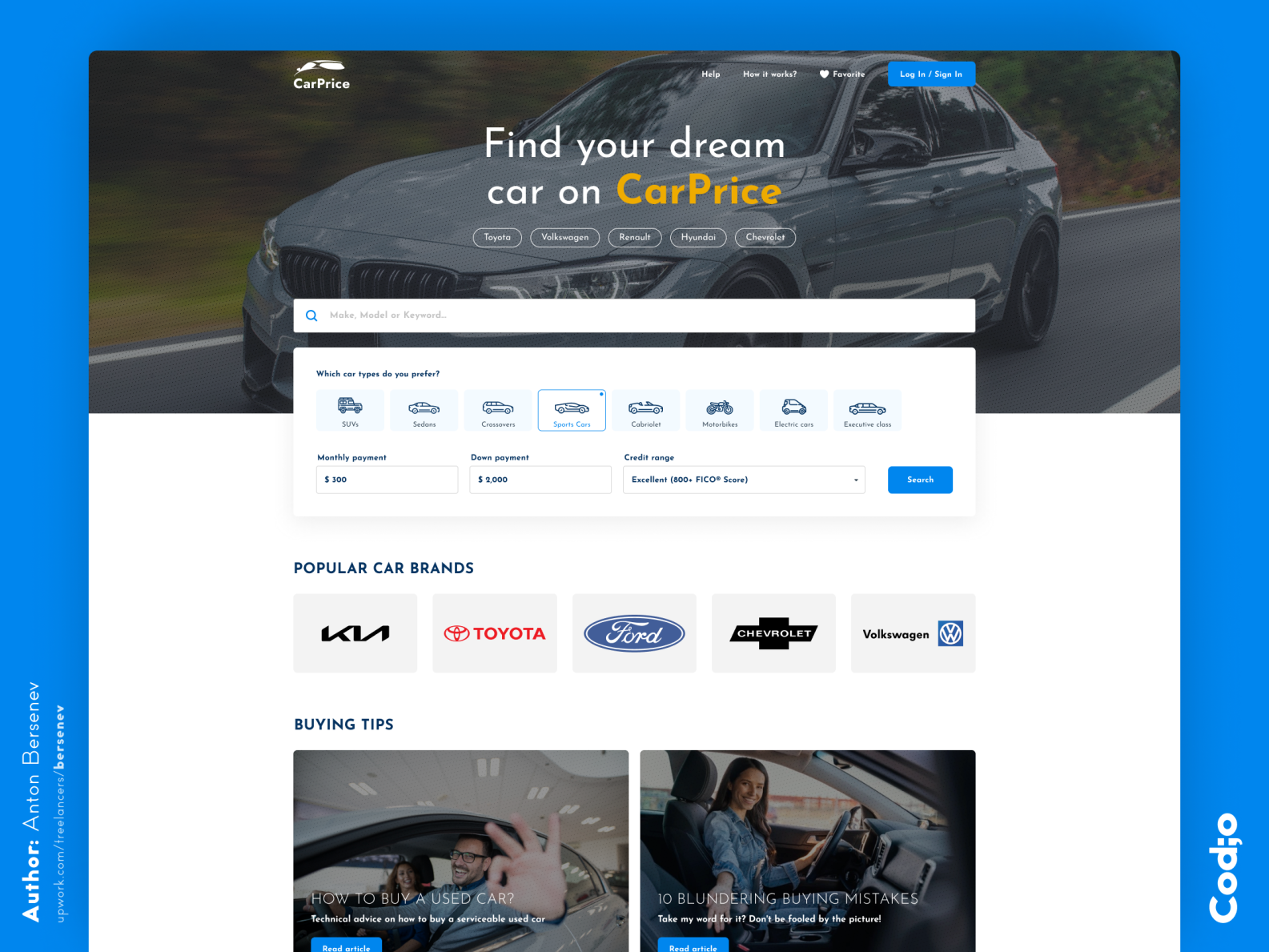This image, sourced from a website, is framed by a blue border on all sides. Within the left-hand side of the blue border, there is a stylized side profile in white, oriented from the bottom left upwards. Adjacent to this profile, also in white text, is the author's name, "Anton Bersenev," written vertically. On the right-hand side of the blue border, again in white text and oriented sideways, it reads "COD, O."

Within this bordered frame, the image contains a central focus: a picture of a dark gray, four-door standard sedan. Positioned above the car, slightly to the left, is the text "Car Price" in white. In the middle part of the image, centered over the car, reads "Find Your Dream Car On," followed by the text "Car Price" in yellow.

Beneath this central image is a series of five clickable white bars, presumably for navigation or selection purposes. Directly below these bars is a white search box equipped with a blue search icon resembling an hourglass. Below the search box is a row featuring eight small icons of cars, although the specific labels beneath them are illegible.

Further down, the image presents three fields for users to input information to specify their desired car type. To the right of these fields, there is a clickable blue box for initiating a search.

Below this search section, a heading in black text reads "Popular Brands." Under this heading, there are five boxes displaying different car brands: Kia, Toyota, Ford, Chevrolet, and Volkswagen.

Next, the section titled "Buying Tips" in black presents two images. The first features a Caucasian couple, with the man in the foreground making an 'okay' hand gesture, and the woman behind him. The second image shows an attractive white woman with brown hair, seated behind the wheel of a car, smiling, and extending her hand towards the camera.